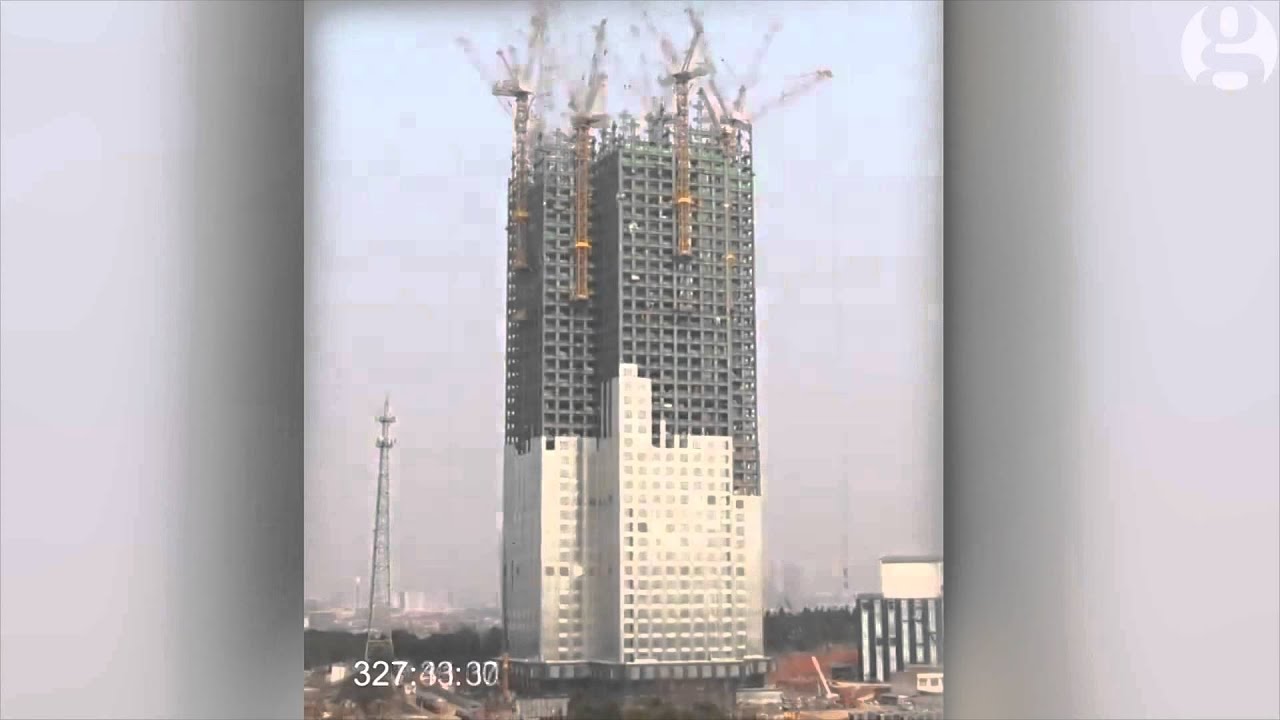The image is a screenshot from a time-lapsed video showcasing the construction of a skyscraper. Displayed in landscape orientation, the main image of interest is in portrait orientation, suggesting it’s a phone screenshot displayed on a computer or laptop. In the top right corner, there is a curvy lowercase "G" watermark, probably indicating the video source. The lower left corner features a timestamp with white numbers reading "327:43:30," though the exact digits might be in motion due to the video’s pause. The skyscraper, characterized by its very tall, rectangular shape with 90-degree angles, is depicted in mid-construction. The lower half of the building already has its white facade, while the upper half remains gray or black, with several cranes actively working on it. Blurry due to the time-lapse pause, the cranes appear to be building the top sections rapidly. Grays, whites, and subtle red accents dominate the muted color palette of the scene.